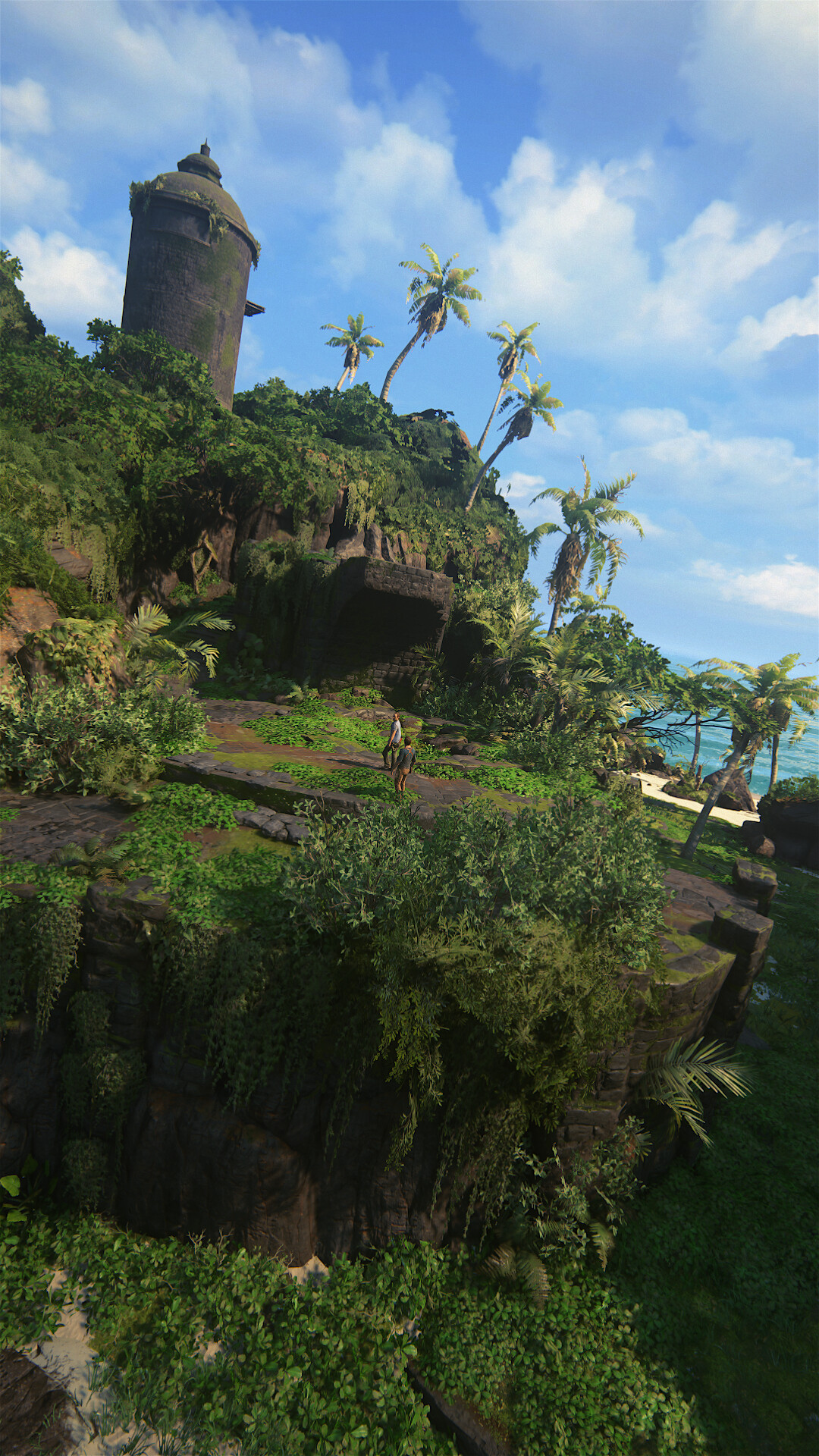This color photograph, possibly generated by AI or part of a video game, depicts a fantastical, somewhat surreal landscape with a clear blue sky dotted with clouds. Situated in the upper left corner is a slightly leaning, round tower. Below it, a lush canopy of palm trees seems to cascade down an edge resembling a mountain or cliff, extending toward a fence on the right side of the image. Under this tower, dense foliage covers a hill that conceals a cavernous opening or cave. Further down in the lower portion of the photograph, additional layers of greenery cloak another cave, with verdant tendrils hanging over its entrance. At the very bottom, more foliage is seen with a prominent shadow on the right side, adding depth and contrast to the scene.